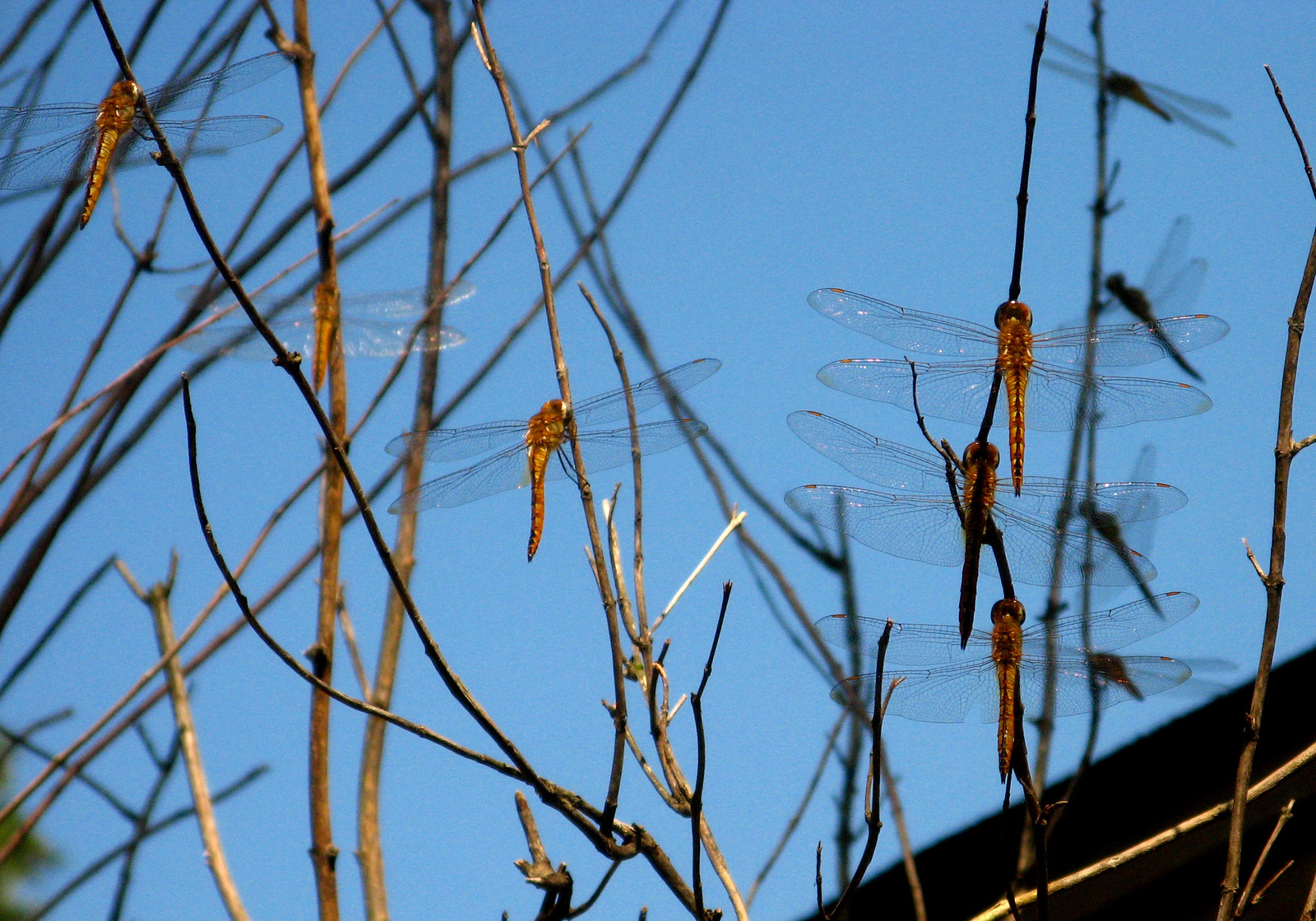This photograph captures a vivid, real-life scene of approximately ten dragonflies interacting with a leafless bush against a bright blue sky. Most of the dragonflies are in close proximity, either hovering or perched on the upward-reaching twigs and branches of the bush, which suggests it might be early spring or late winter. In the foreground, six dragonflies are clearly visible, showcasing their slender, light brown bodies and distinct four transparent wings. Their elongated bodies are bulbous at the head, tapering to a pointed tail, with prominent eyes that stand out in the image. In the top right corner, a roof structure from a distant building is partially visible, adding a subtle architectural element to the natural setting. Additionally, a tiny hint of green vegetation can be seen, slightly blurred, in the bottom left corner of the photograph.